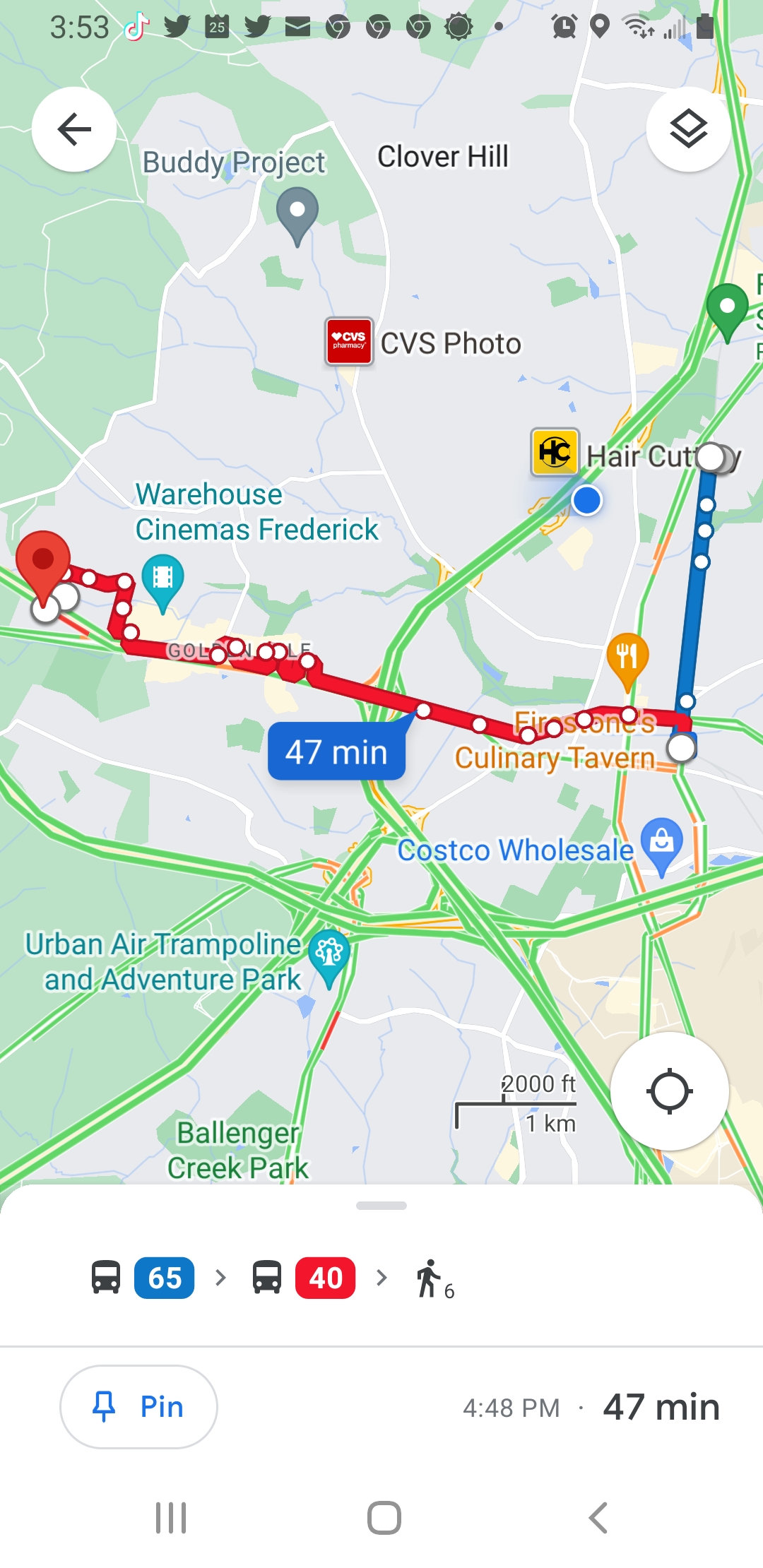This image is a detailed, color screenshot of an iPhone displaying Google Maps directions for a route in the United States. The map is vertical and prominently features a red line indicating the path from the starting location to a destination, which appears to be a hairdresser or hair cutter. The trip will take a total of 47 minutes and requires taking the 65 bus followed by the 40 bus, and then a 6-minute walk. Landmarks such as CVS, CVS Photo, Costco, Clover Hill, Buddy Project, and Ballinger Creek Park are marked along the route. At the top, the time is displayed as 3:53, and various app icons, including Chrome and TikTok, can be seen. Additionally, there's a small key at the bottom of the map indicating distances in feet and kilometers. The lower part of the screen shows symbols for bus routes and walking directions, with a clickable button offering further options.